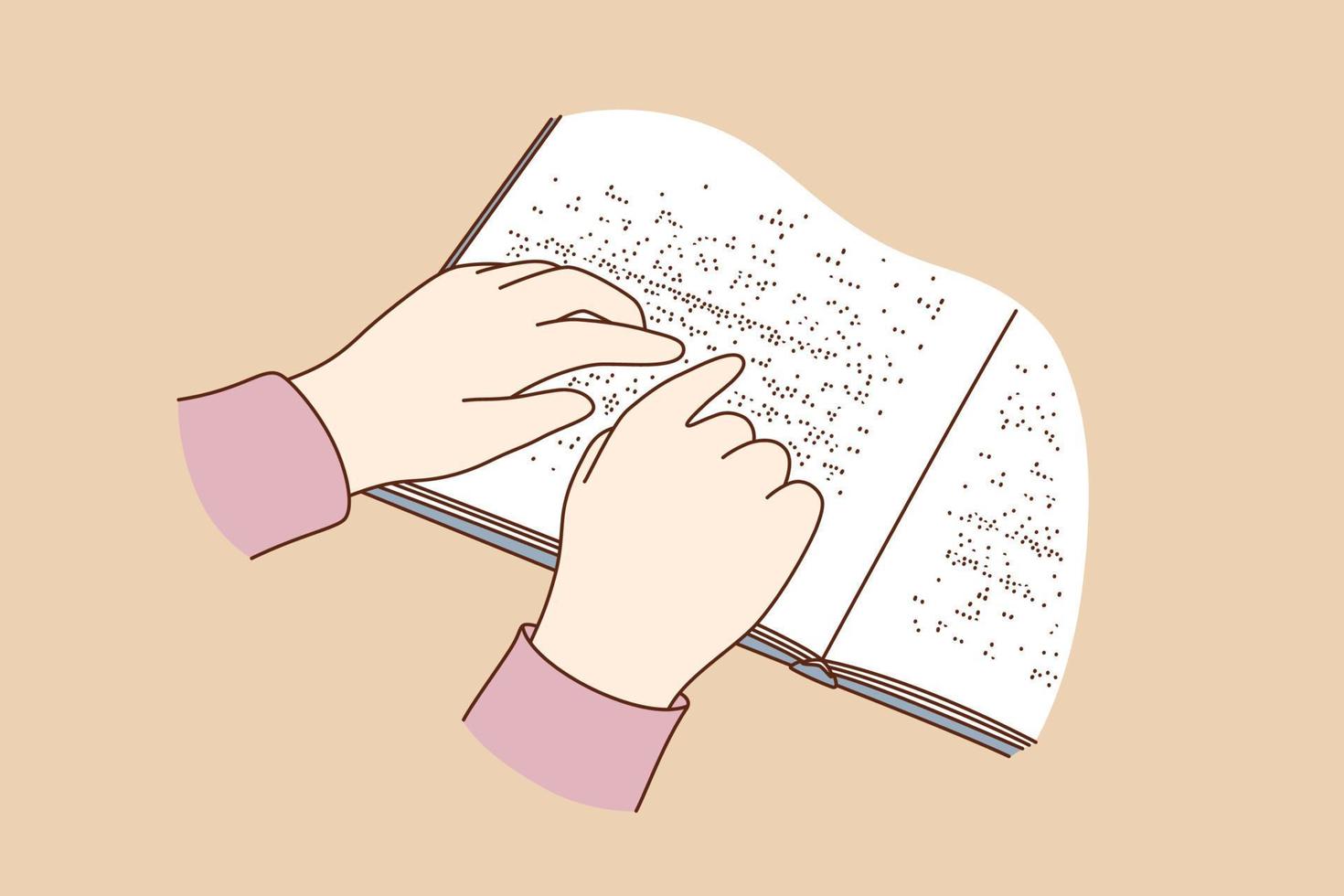This image depicts a digitally illustrated scene of a woman reading a braille book against a dark cream-colored background. The rectangular image, which is wider than it is tall, centrally features an open braille book that is partially cropped at the top and the right-hand side, displaying predominantly the left-hand page. The pages are white with raised black specks representing the braille text. The woman’s hands, which are a light brown with slight pinkish tones and outlined in black for distinction, are placed on the braille text, indicating that she is actively reading it. The woman is wearing a maroon and purple-hued sleeve that covers her wrists visibly. The hands originate from the bottom left of the scene, maintaining their position in the center of the image. The overall style of the artwork appears to be a digital painting, creating a vibrant and detailed visual of a tactile reading experience.